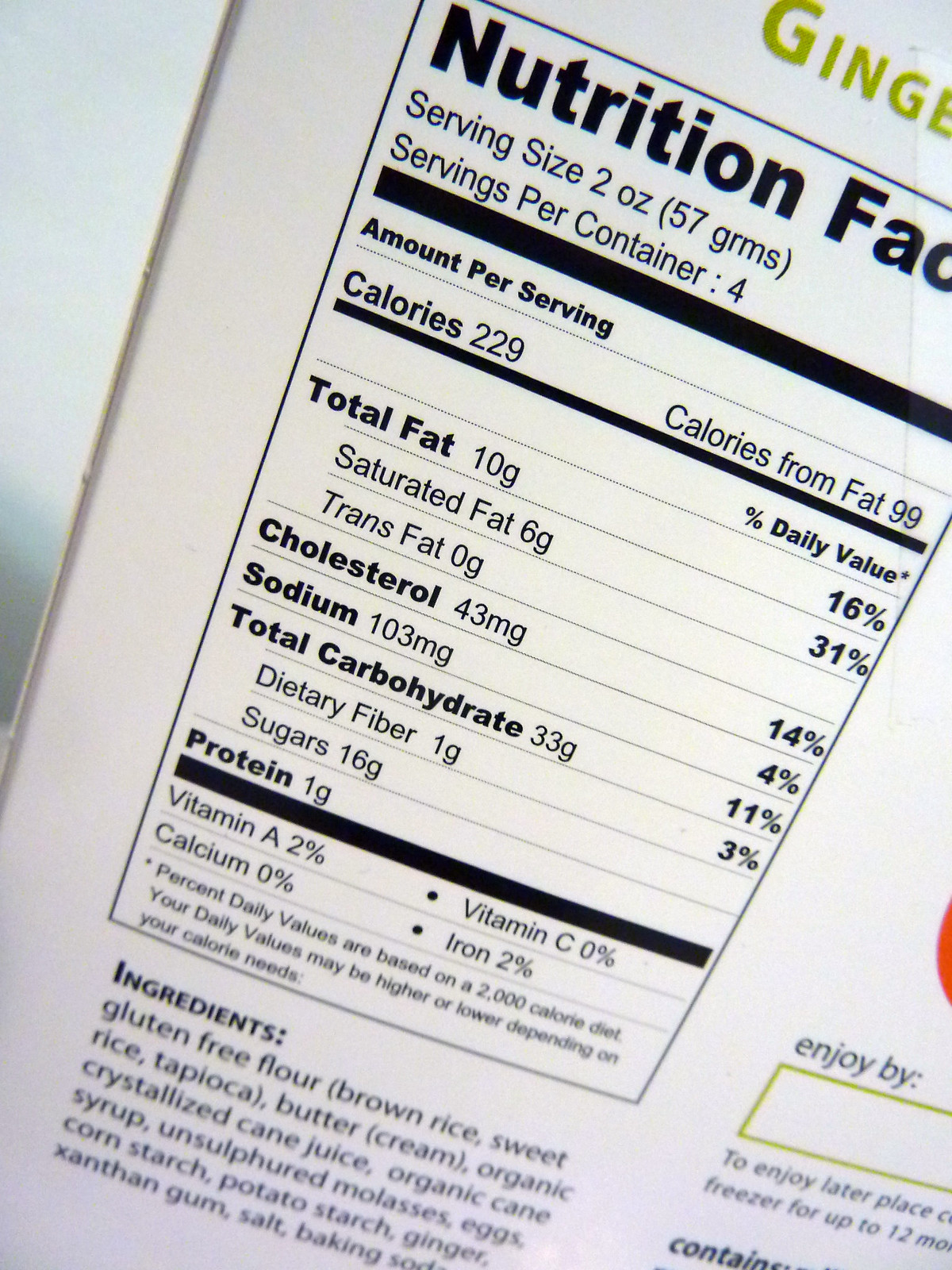This is an up-close photograph of a Nutrition Facts label on a white box, which is positioned at an angle to the right. The box features a light blue upper left-hand corner that transitions into a darker blue towards the bottom. Prominently displayed in green text at the top right corner are the partially cut-off letters "GINGE," likely indicating "Ginger." Below this, the bolded "Nutrition Facts" title stands out in black. The label details a serving size of 2 ounces (57 grams) with 4 servings per container. Each serving contains 229 calories, 10 grams of total fat (including 6 grams of saturated fat), 43 milligrams of cholesterol, 103 milligrams of sodium, 33 grams of total carbohydrates (with 1 gram of dietary fiber and 16 grams of sugar), and 1 gram of protein. Additionally, the product provides 2% of the recommended daily value for Vitamin A and iron. The ingredients listed at the bottom include gluten-free flour, brown rice, sweet rice, butter, cream, organic crystallized cane juice, organic cane syrup, unsulfured molasses, eggs, corn starch, potato starch, ginger, xanthan gum, salt, and baking soda.